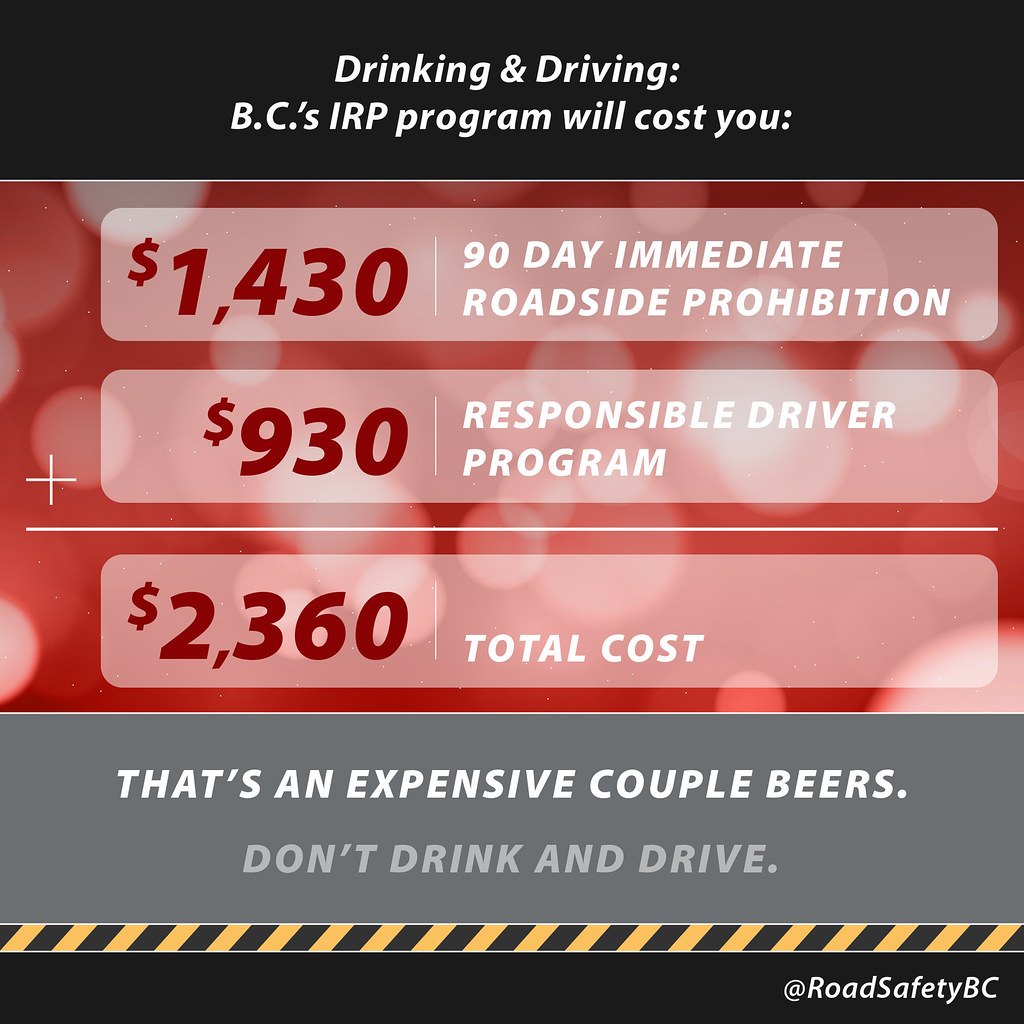The image appears to be an informational slide about the costs associated with drinking and driving under BC's IRP program. The slide is divided into four distinct sections. The top section features a black background with white text that reads, "Drinking and Driving, BC's IRP program will cost you." Below this, the central portion has a red background with pink dots, displaying three lighter red rectangles with red and white text. This text itemizes the costs as "$1,430 for a 90-day immediate roadside prohibition," and "$930 for the responsible driver program." A math line underneath these amounts shows their addition, culminating in "Total Cost: $2,360."

The bottom section has a gray background with white and light gray text, stating, "That's an expensive couple beers, don't drink and drive." A small caution banner with a yellow and black design appears at the very bottom. Finally, in the bottom right-hand corner, there is a black section with white text that reads, "At Road Safety BC." The overall image is vivid and clear, utilizing a color palette that ranges from black and white to various shades of red, gray, and yellow.